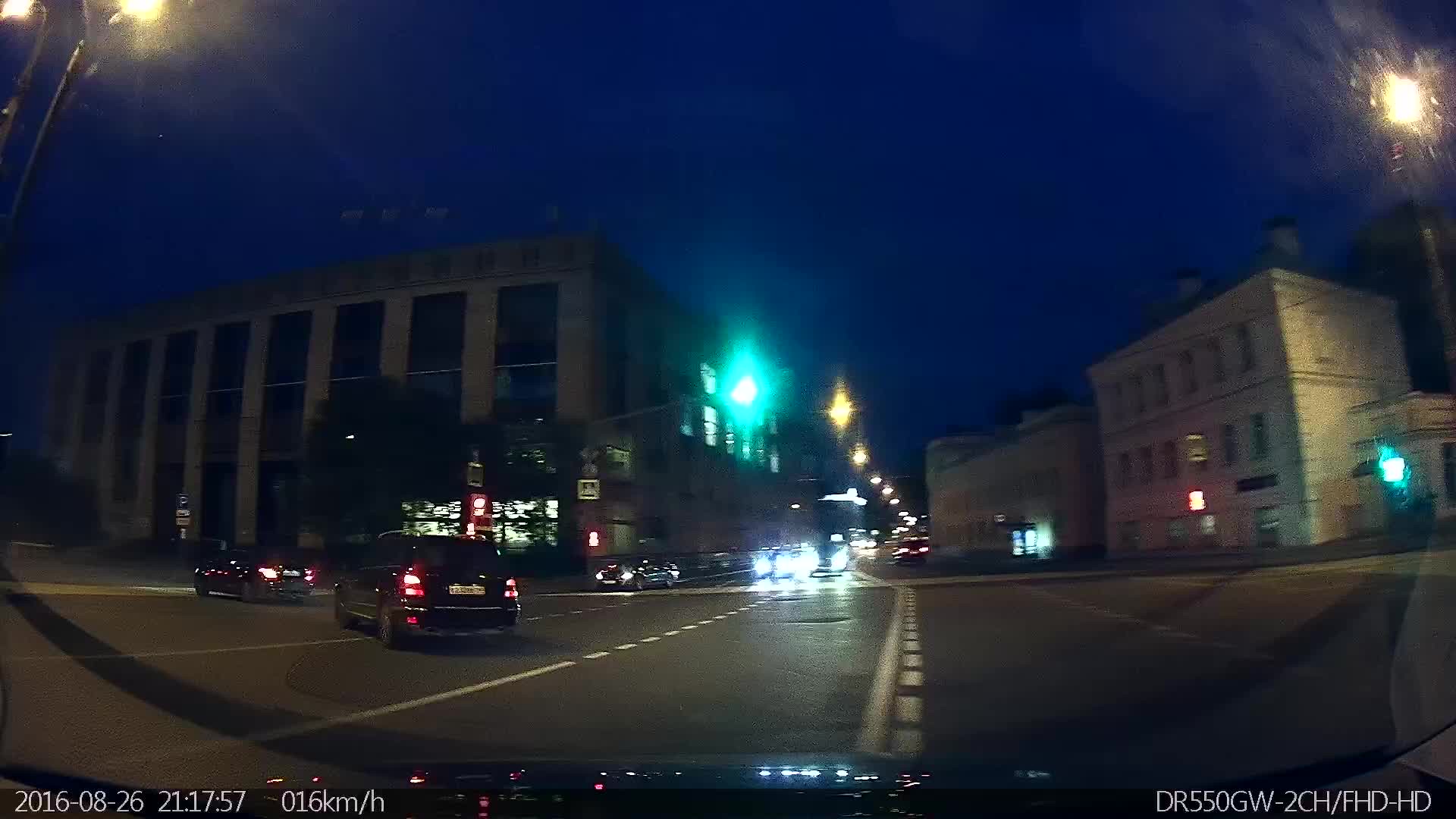A vivid nighttime traffic scene is captured, set against a backdrop of a dark blue sky. Dominating the right side of the photo is a three-story building featuring gray sections between each floor and at the roofline, which separates the windows. The building's gray top extends to about half the height of the windows below it. In the foreground, the street is bustling with activity as two cars, a minivan, and a sedan, are visible making a right turn, effectively turning to their left from our perspective. Their taillights glow brightly, adding to the nocturnal ambiance. In the distance, oncoming headlights pierce through the darkness, indicating traffic moving towards the camera. Adjacent to the three-story building, a green traffic light, clearly visible, directs the flow. Further to the left stands a two-story building with six evenly spaced windows. Yellow traffic lines on the road delineate lanes, adding structure to the nighttime scene.